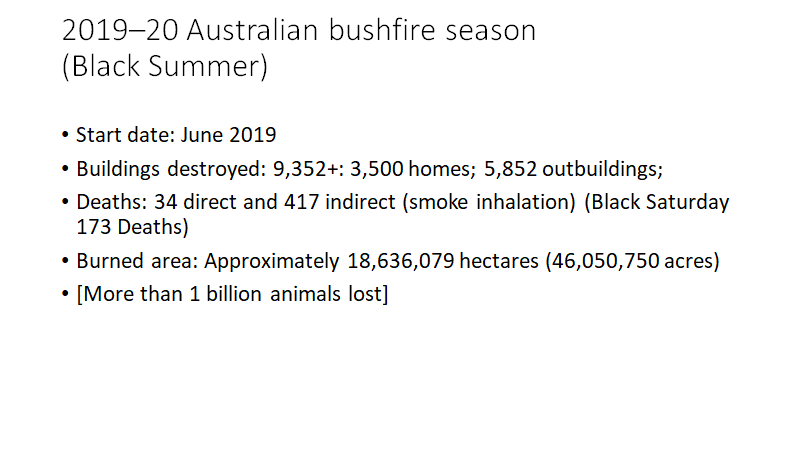**Descriptive Caption: Australian Bushfire Black Summer 2019-2020**

The image encapsulates a detailed overview of the devastating Australian bushfire season, often referred to as the "Black Summer" of 2019-2020. The caption is laid out on a plain white background with black text, featuring prominent detailing:

- **Title:** "2019-2020 Australian Bushfire Season (Black Summer)"
  - The title is slightly larger and bolder compared to the other text elements.
  
- **Details:**
  - **Start Date:** June 2019
  - **Destruction:** Over 9,352 buildings destroyed, including:
    - 3,500 homes
    - 5,852 additional structures (referred to as outbuildings)
  - **Human Impact:**
    - 34 direct fatalities
    - 417 indirect fatalities due to smoke inhalation
    - A reference to the tragic Black Saturday event with 173 deaths
  - **Burn Area:** Approximately 18 million hectares (46 million acres)
  - **Wildlife Impact:** Over 1 billion animals lost

This image highlights the sheer scale of the disaster, both in terms of the human tragedy and the massive environmental impact. In addition to the stark factual data, a personal anecdote is linked to the image, recalling how a bodybuilder, originally from Australia, returned from California to assist his family during the wildfires. The simplicity of the black-on-white text format underscores the seriousness and gravity of the information being presented.